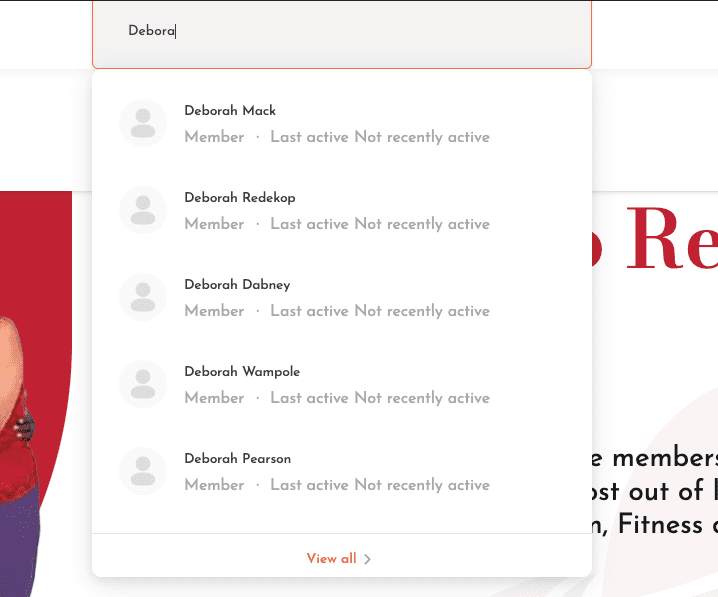In this image, a pop-up search bar is prominently displayed in the foreground, obscuring portions of the background which features red images and text. The search bar is situated at the top of the window, and it appears that a user has started typing the name "Deborah." Below the search bar, a list of search results is visible, each entry consisting of a name, a member status, and their last active status, all indicating "not recently active."

1. "Deborah Meck" - Member, last active: not recently active.
2. "Deborah Readycup" - Member, last active: not recently active.
3. "Deborah Dabney" - Member, last active: not recently active.
4. "Deborah Wampole" - Member, last active: not recently active.
5. "Deborah Pearson" - Member, last active: not recently active.

At the bottom of the search results, there is an option highlighted in red that reads "View All."

This detailed caption paints a clear picture of a user interface element listing various members named Deborah, none of whom have been recently active.